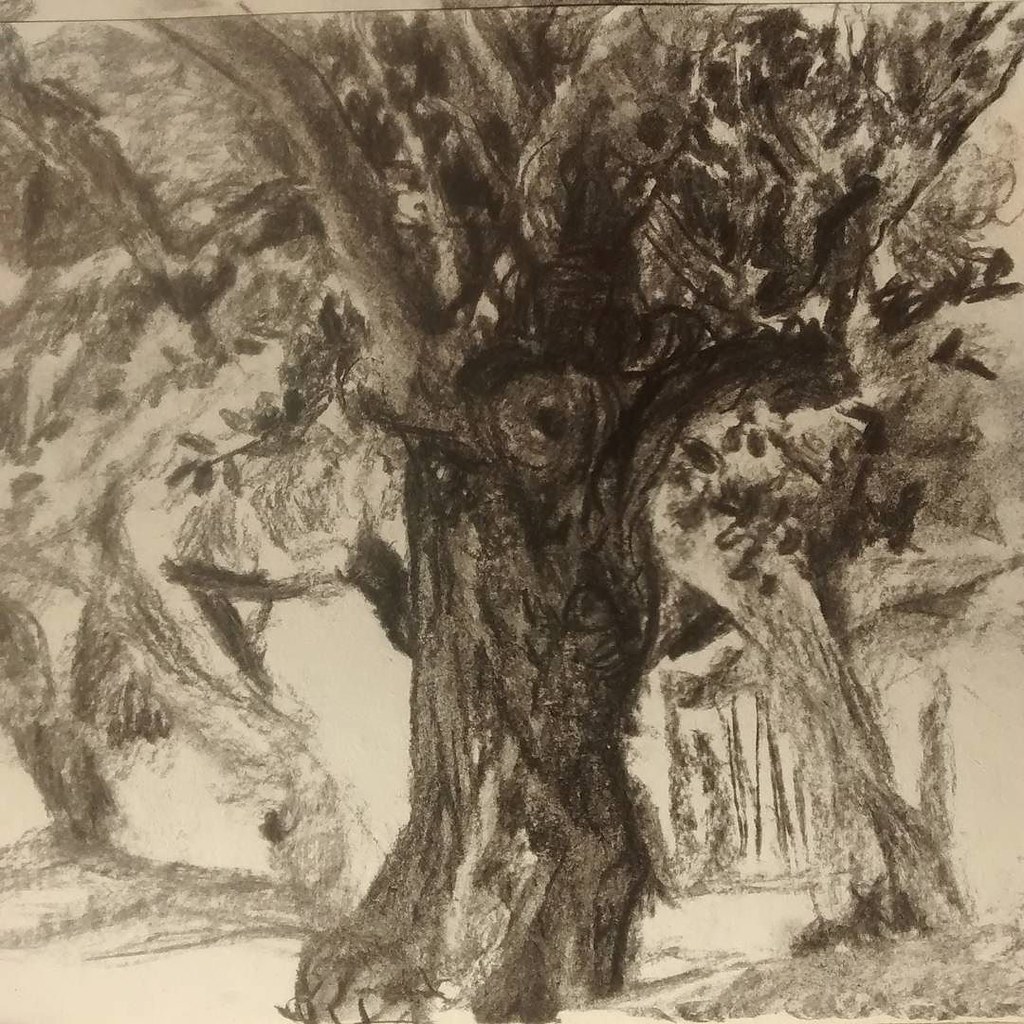The image depicts a detailed pencil drawing on yellowish paper, showcasing a large, prominent tree as its focal point. The tree features a thick, deeply textured bark leading down to the bottom, with a significant knot at its center. Its branches extend outward, with the left side appearing somewhat bare while the right side is lush with leaves. Surrounding the main tree are outlines of several other trees with branches and leaves, contributing to a woodland scene. To the right of the tree, there is a noticeable tree stump, and to the left, a round structure with a small black shape within it. In the background, finer details suggest additional smaller, skinnier trees and the hint of a path running through the woods, adding depth to the composition and enhancing the woodland atmosphere.